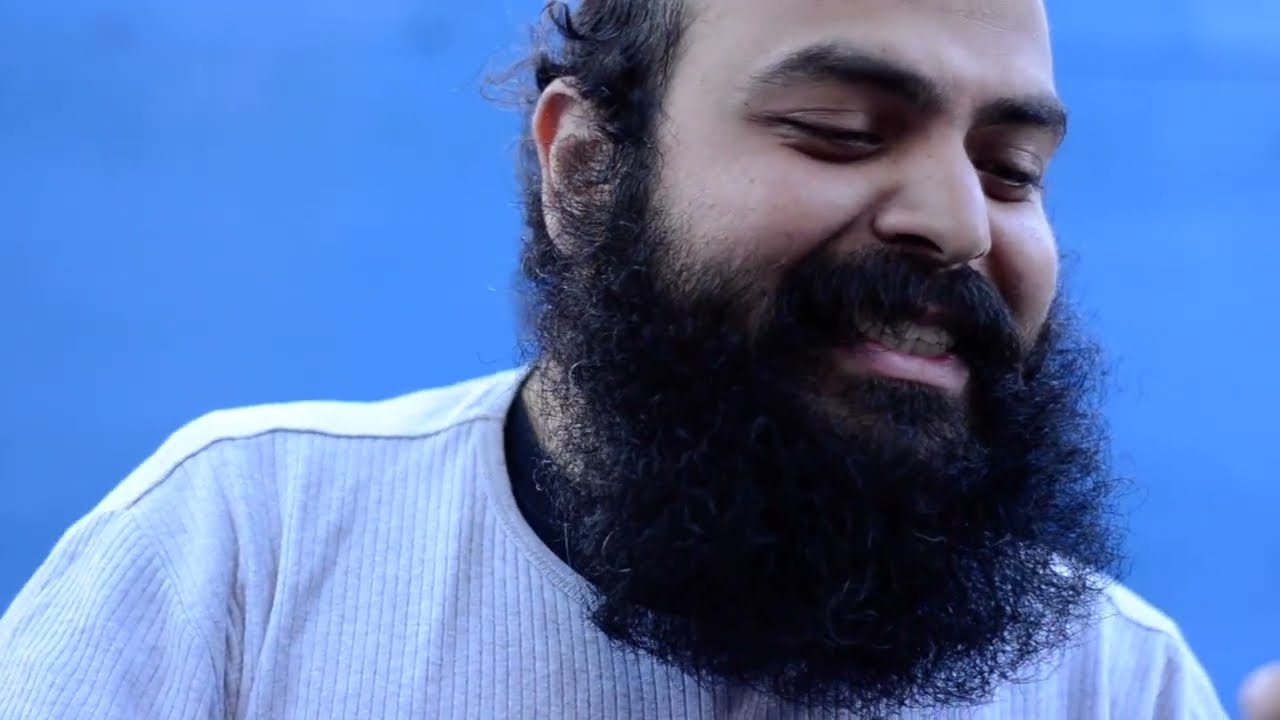In this outdoor daytime photo, a man with olive skin, dark hair, and a long, curly dark beard and mustache is seen from a side angle, occupying the left side of the frame. He is wearing a white t-shirt over a black shirt, with the black collar visible under his beard. His eyes appear closed or tightly squinted. He is holding a cell phone in his left hand while gesticulating with his right, perhaps during a video call. The background features a pale blue concrete wall and some tree branches visible at the top right, set against a bright, glary white sky. The image captures the man mid-conversation, with his expressive gestures adding a dynamic element to the scene.